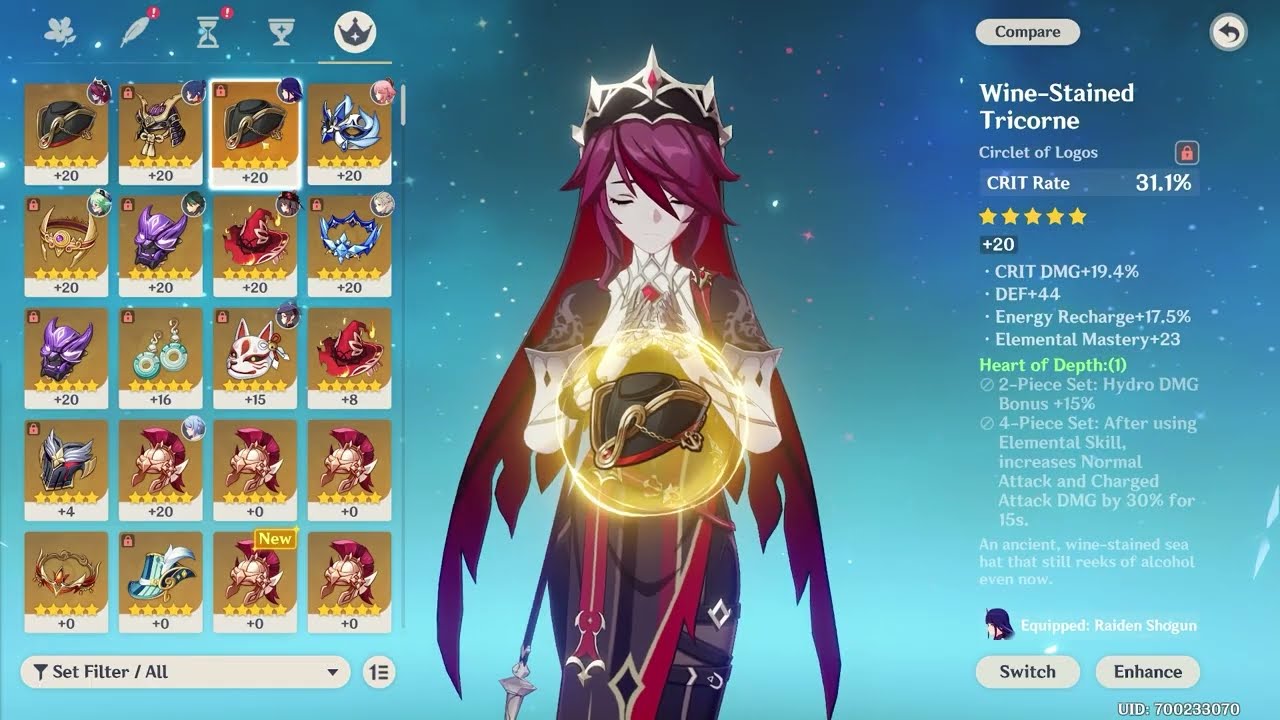This screenshot from a computer or mobile application game features a horizontally rectangular interface with a dark-to-light blue sky background, scattered with tiny white stars. Dominating the center is an animated woman with shoulder-length, maroon-pinkish purple hair, which covers her arms. She wears a black and silver crown, has her eyes closed, and holds a yellow orb encased in a gold device in front of her as if praying. Her attire includes long purple and dark pink robes, giving her a mystical, wizard-like appearance.

To the left, the interface displays a grid of 20 symmetrically aligned character icons in four columns and five rows, depicting various creatures. Beneath this grid, there's a white button labeled "Set Filter / All.” Above these icons, three gray outlines of an hourglass, a trophy, a leaf, and a flower are visible, with the crown icon currently active.

On the right side, the screen provides detailed information about the selected item, labeled "Wine Stained Tricorn" and "Circlet of Logos." Its attributes are listed, including "Crit Rate 31.1%,” accompanied by five yellow stars and a "+20" notation. Beneath this, a descriptive paragraph offers additional game-specific information. Two white buttons, "Switch" and "Enhance," are located at the bottom right. Above this section is a small, curved left arrow labeled "Compare Button," facilitating navigation back to previous menus.